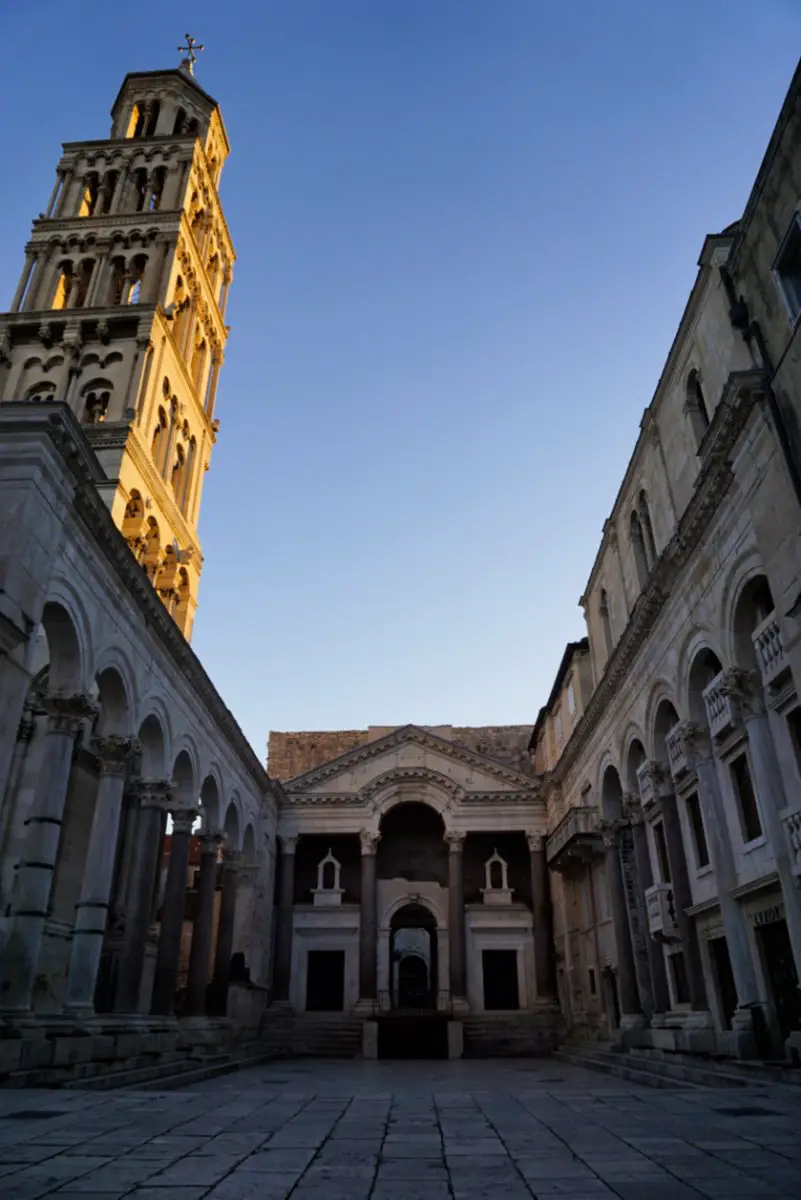The image captures an extensive and elaborate ancient building, likely a church, with a distinctly Spanish architectural influence. A clear, blue sky without any clouds frames the background, with sunlight illuminating the tall steeple and spire on the left side of the structure. This steeple features a cross at the top and consists of four ornate layers adorned with intricate filigree and archways. The photograph is taken from a street-level perspective, making the towering structure appear even more imposing.

Flanking the central courtyard are large stone arches—about seven on each side—that lead up to columns, giving the impression of a space surrounded by the building's grandeur. The courtyard ground is made up of dark gray bricks, adding a stark contrast to the light tan or off-white color of the buildings. Shadows dominate the courtyard, while the main building front and the steeple are highlighted by the sunlight.

The entrance to the central structure is characterized by a large archway flanked by two smaller rectangular doorways. Stone steps are visible on either side, ascending to additional arches and columns. Through these large open arches and windows, one can see a glimpse of the blue sky, emphasizing the openness and scale of the architecture. The perspective suggests standing in the middle of a square walkway, surrounded and overshadowed by the immense, majestic construction.